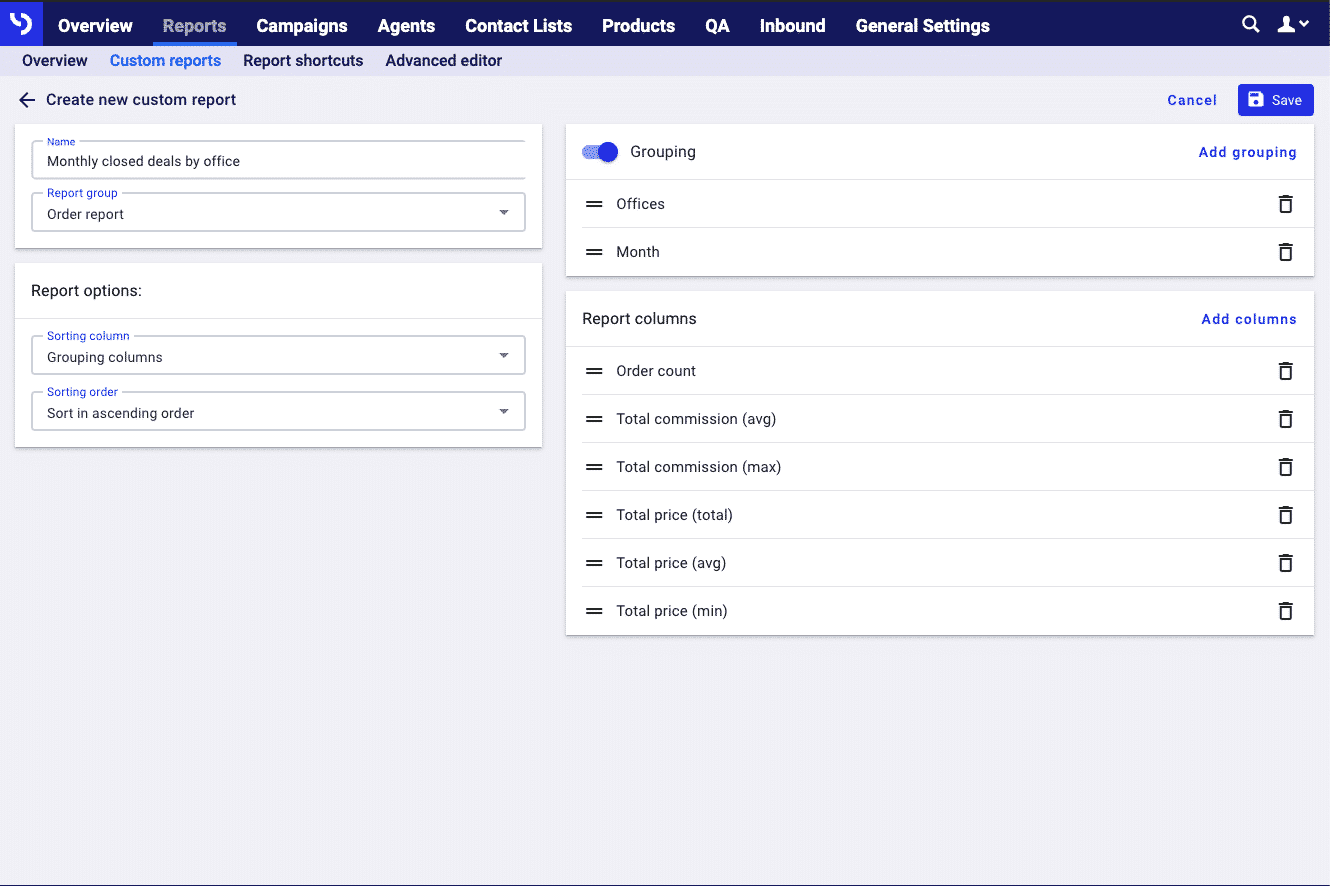The web page is set against a very pale blue background. At the top of the page, a navy blue banner spans horizontally across the screen, featuring several navigational options in white text: Overview, Reports, Campaigns, Agents, Contact Lists, Products, QA, Inbound, and General Settings. To the right of these options, there are icons for a magnifying glass, a people icon, and a down arrow.

Beneath this main banner is a thinner, slightly darker blue banner with navy blue text on the left displaying: Overview, Custom Reports, Report Shortcuts, and Advanced Editor. The "Reports" and "Custom Reports" options are currently selected.

In the main content area, large navy text indicates "Create New Custom Report" accompanied by a back arrow. Below this title is a white box containing two fields labeled "Name" and "Report Group." The "Name" field is filled with "Monthly Closed Deals by Office" and the "Report Group" field contains "Order Report."

Further down, another white box labeled "Report Options" is present, containing additional customizable settings. 

The page appears to be part of an application for generating and managing custom reports, providing a clear and organized interface for the user to create and categorize their reports.